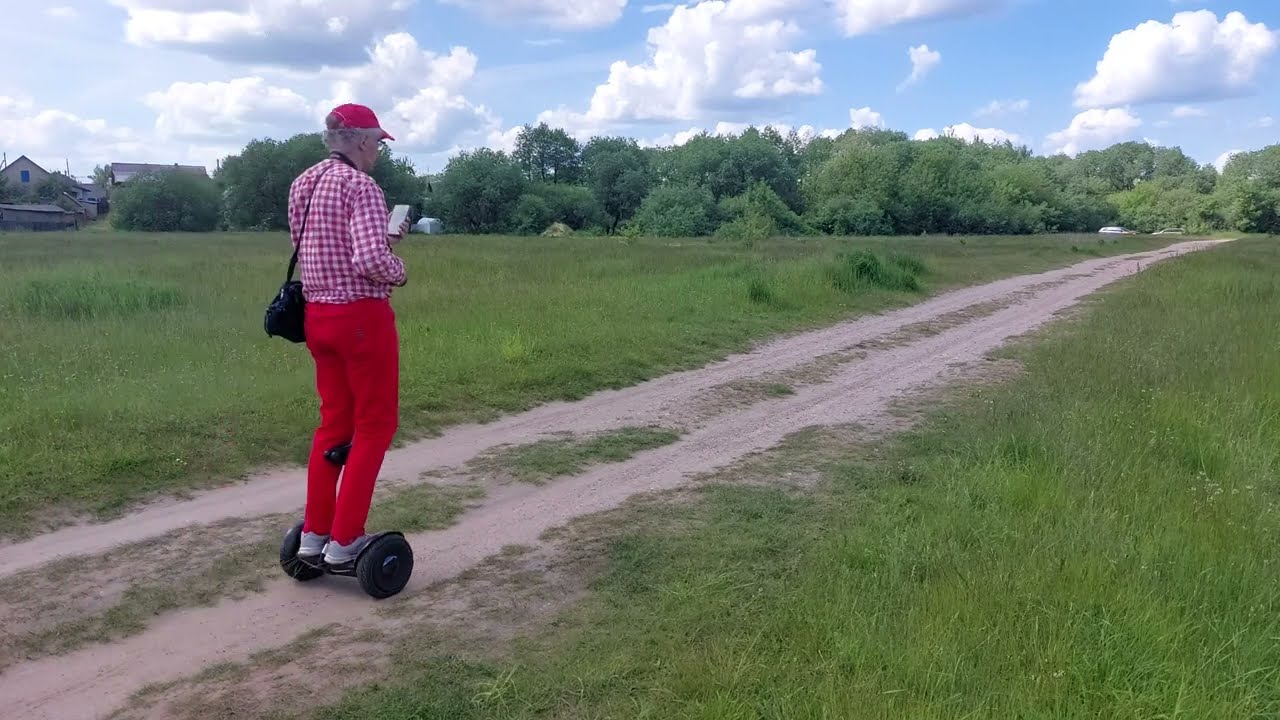The landscape-oriented color photograph depicts an elderly individual, distinguishable by their glasses and eccentric attire, riding a black hoverboard along a dirt path in a rural setting. The path, starting from the bottom left and extending towards the top right, is flanked by green grass and leads to a distant field of trees. On the left side of the image, a couple of buildings can be seen under a blue sky dotted with puffy white clouds. The elderly individual, centrally positioned yet slightly left-leaning, wears red pants, white sneakers, a red baseball cap, a checkered red and white shirt, and a black belt bag slung over their left shoulder. They hold a smartphone in their left hand, seemingly absorbed in it. The scene exudes a quiet, small-town ambiance in the middle of the day.